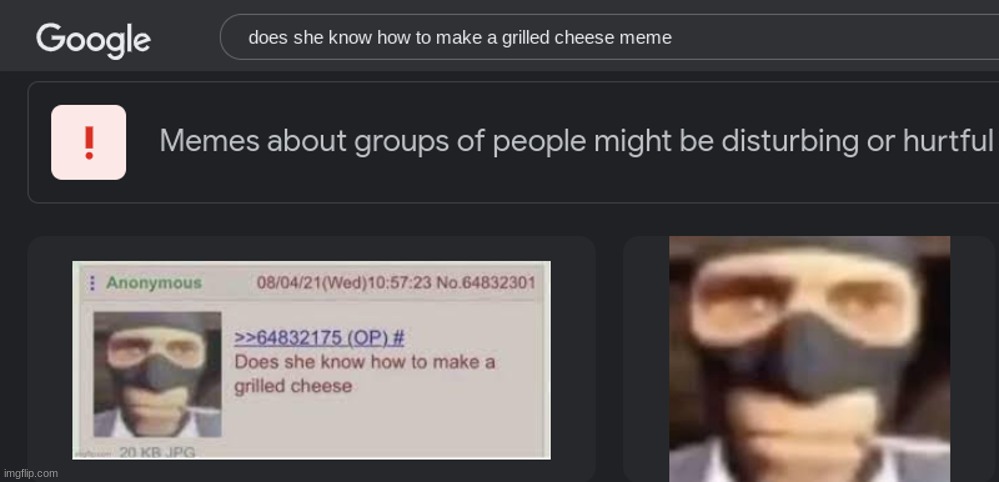**Detailed Caption:**

The image is a long horizontal rectangle with a black background, adorned with white text and various pictures. In the upper left corner, the word "Google" appears in white letters. Below it is a search bar containing the query: "does she know how to make a grilled cheese meme". 

Beneath the search bar, there is a white box with a red exclamation point inside. This box contains a warning that reads: "Memes about groups of people might be disturbing or hurtful."

In the lower left of the image, a gray rectangle is displayed. In the upper left of this rectangle, the word "Anonymous" is written in green. To the right of "Anonymous," the date "8/4/21" is shown in red, followed by "Wednesday" and the time. 

Below "Anonymous," there is a picture of a man wearing a black mask which covers his head, nose, and cheeks, leaving only his eyes, mouth, and lower chin visible. His expression appears menacing, with a very straight mouth, a square chin, and stern-looking eyes.

To the right of the masked man's image, the text reads: "Does she know how to make a grilled cheese." 

The same image of the masked man is repeated in the bottom right of the image. This version is a closer, albeit blurrier, depiction of the man's face. The cropped, magnified image highlights the same menacing features, adding to the overall eerie feel of the image.